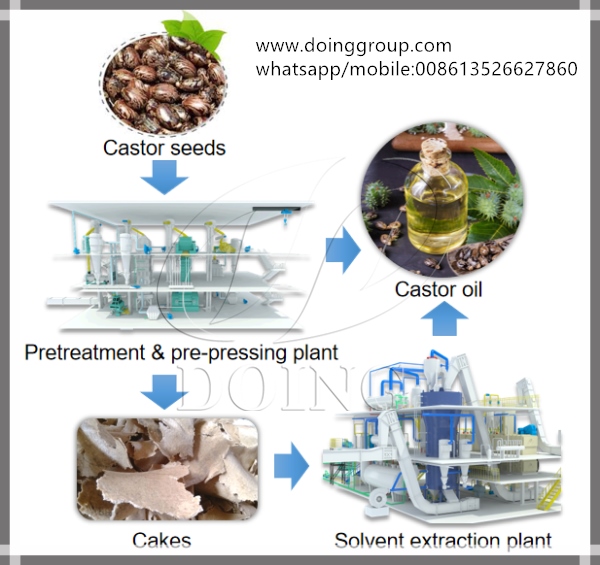This descriptive image, likely an indoor infographic, presents the process of castor oil extraction within a bordered white square. The gray border frames a composite of images and text illustrating the sequence. At the upper right corner, the URL www.doinggroup.com is displayed along with "WhatsApp/mobile: 00861-352-6627-860." On the upper left, a circular image portrays brown castor seeds, captioned "castor seeds" in black text. A blue arrow points downward to an industrial facility labeled "pretreatment and prepressing plant," depicting green and gray cylindrical machinery. From this plant, the process branches out; a blue arrow leads to the right to a blue and silver metallic "solvent extraction plant" with prominent pipes, above which another blue arrow directs upwards to an image of a jar labeled "castor oil." Meanwhile, a downward arrow from the pretreatment plant points to an image of rectangular brown shapes labeled "cakes," which also connects rightward to the solvent extraction plant. The bottom section of the infographic includes the faint white text "DOING," with the tail of the "G" overlapping slightly into the solvent extraction plant image.